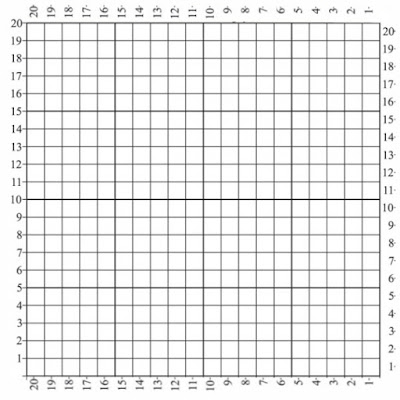The image depicts a detailed grid with dimensions of 20 by 20 squares, all lines rendered in black with the overall background being light blue. Each side of the grid is meticulously numbered from 1 to 20. The left side is numbered ascendingly from 1 at the bottom to 20 at the top, while the right side follows the same format. Conversely, the top edge numbers descend from 20 on the left to 1 on the right, and the bottom edge mirrors this sequence from 20 on the left to 1 on the right. Notably, the grid features a central horizontal line, situated between the 10th and 11th rows, which is distinguished by being bolder and darker than the other lines. This visual detail accentuates the symmetry and precise layout of the graph, although the interior squares remain empty, devoid of any additional markings or data.